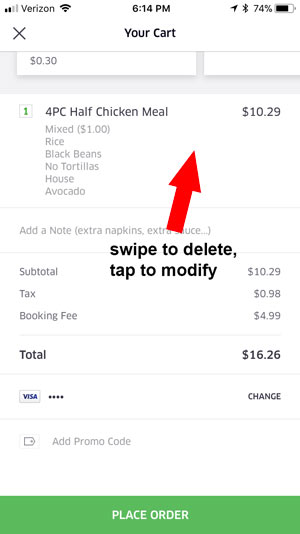The image is a screenshot of a mobile checkout page for a food order, taken on a Verizon cell phone at 6:14 PM with a battery level of 74%. At the top of the screen, it displays "Your cart" with an option to exit marked by an 'X'. The cart contains one item:

- 4 PC Half Chicken Meal priced at $10.29.
- Below, it specifies the meal details: "Mixed $1 rice, black beans, no tortillas, house avocado."
- There is also an "Add a note" section, where "extra napkins" and "extra sauce" have been requested.

The subtotal for the order is $10.29, with an additional tax of 98 cents and a booking fee of $4.99, bringing the total to $16.26. The payment method is listed as Visa, with an option to change the card information. There's also an area to add a promo code.

At the bottom of the screen, a green rectangle with white text reads "Place Order". A red, thick arrow pointing upwards is in the middle of the page, overlaid with black text that says "Swipe to delete, tap to modify".